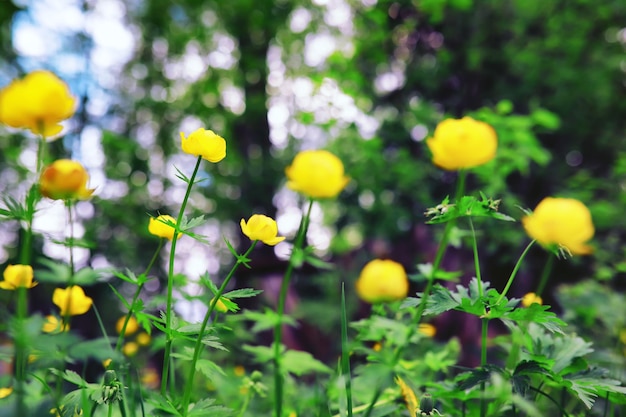The image is a horizontally aligned, slightly blurry photograph capturing a close-up of around 10 to 12 small, yellow, bulb-shaped flowers with long, thin green stems and parsley-like leaves, set against a grass-covered foreground. The yellow flowers at the center and slightly off to the left are in focus, revealing delicate petals, while the others appear as blurred yellow circles. The background is densely filled with green leaves and trees, with patches of blue and purple light filtering through the foliage. Small white dots, which might be the sky shining through the leaves, add to the depth of the image, particularly noticeable at the upper left.